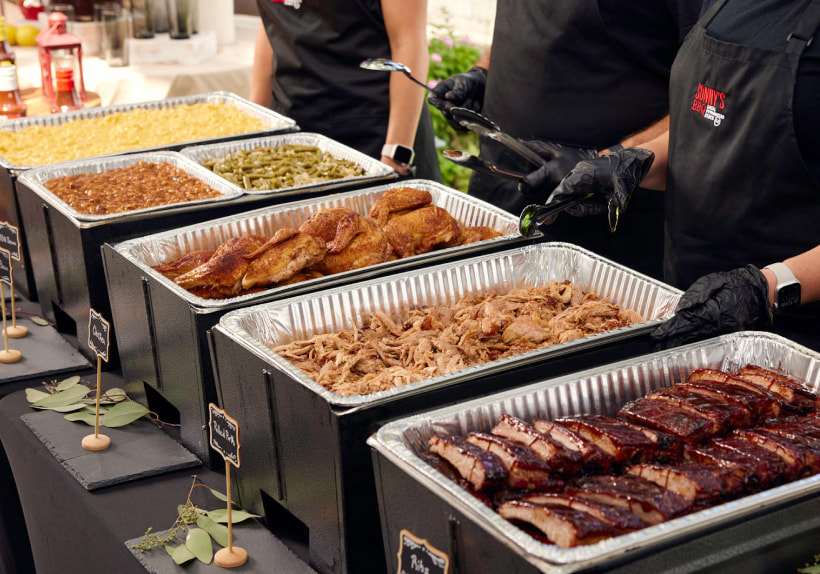The image depicts a close-up view of a buffet table lined with an array of food trays. The black rectangular holders, each containing an aluminum tray, measure approximately one foot by two and a half feet and are around 10-12 inches deep. Placed in these trays, a selection of various dishes is visible, notable among which are cuts of beef, fish, corn, green beans, and perhaps macaroni and cheese. In front of each tray, there are small wooden stands with black rectangular signs displaying off-white text, though the specific labels are unreadable.

Behind the buffet stand three employees, dressed uniformly in black attire that includes aprons and gloves. Notably, the individual on the right is adorned with a black shirt and an apron that features the red emblem of Sunny's Barbecue. Their faces and lower bodies are out of the frame, emphasizing their midsections as they prepare to serve food. Two of them wield tongs, with one also clutching a ladle, ready to assist the guests. The scene captures a moment of poised service amidst a well-organized buffet setup.